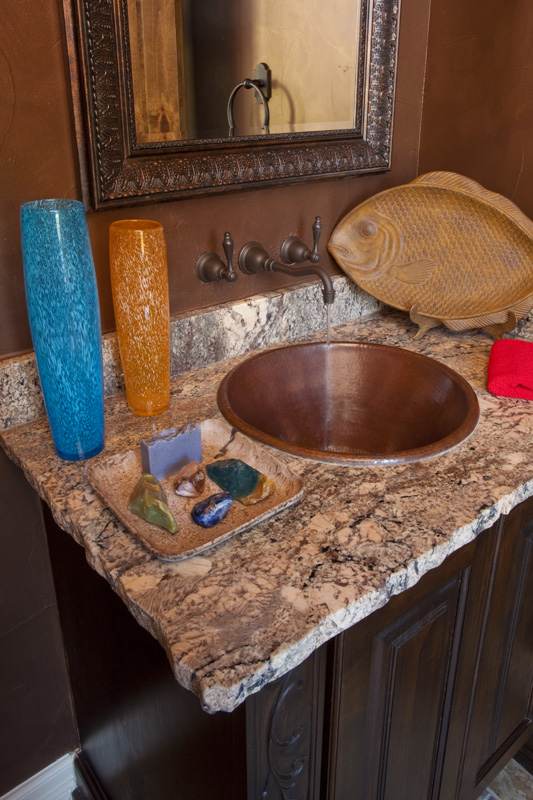The image showcases a wash hand basin elegantly integrated into the corner of a room. The walls are painted a deep, rich brown color, complementing the matching deep brown wooden cabinet that supports the basin. The countertop features a striking marbled pattern in shades of white, black, and brown, harmonizing perfectly with the overall color scheme.

The wash hand basin itself is a unique brown hue, blending seamlessly with the wall and cabinet. Atop the countertop sits a decorative blue and orange jug, adding a pop of color to the earthy tones. Positioned in the corner of the counter, a decorative brown fish ornament enhances the aesthetic appeal. Scattered beside the basin are colorful stones in varying shades of blue, green, and brown, contributing to the decor’s natural and artistic vibe.

Above the wash hand basin, a piece of wall art is displayed, further enriching the visual interest of this stylish and meticulously designed corner.